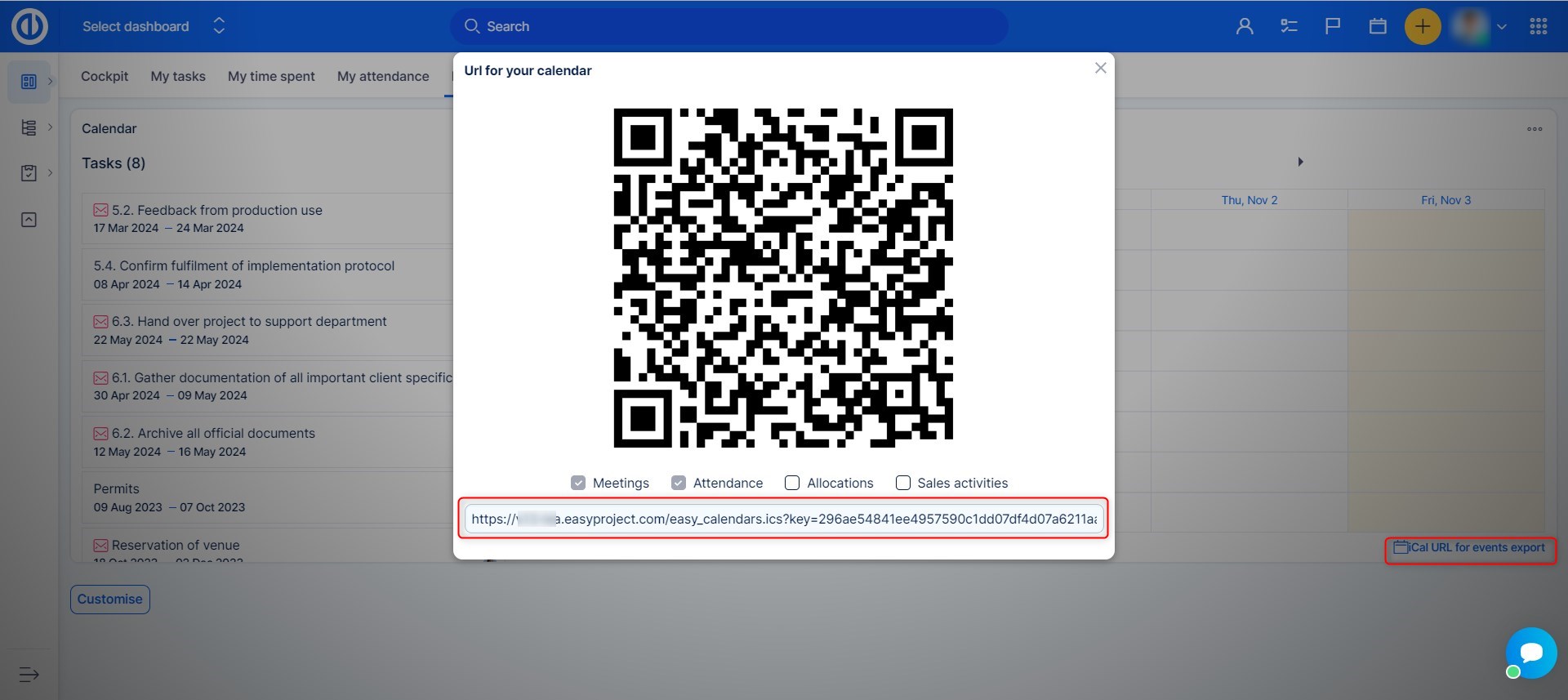The screenshot from a website features a prominent QR code pop-up in the foreground, designed for users to scan and access a URL related to calendar features. The text on the pop-up reads "URL for your calendar." Beneath the QR code, the website URL has been intentionally blurred, yet it is outlined in a red rectangle, likely for instructional emphasis. 

In the background, there is another red rectangle surrounding the text "CAL," which is an abbreviation for calendar, accompanied by a calendar icon. Adjacent to this, it indicates "URL for events export." Although the background is muted and harder to discern due to the pop-up, a closer look reveals a large blue rectangle at the top labeled "Select Dashboard." This area includes a search bar, a blurred profile picture for privacy, and a nearby yellow circular icon featuring a plus sign. Additionally, the interface shows options such as "Calendar" and "Tasks," with a task count of eight and a detailed list of tasks below this section.